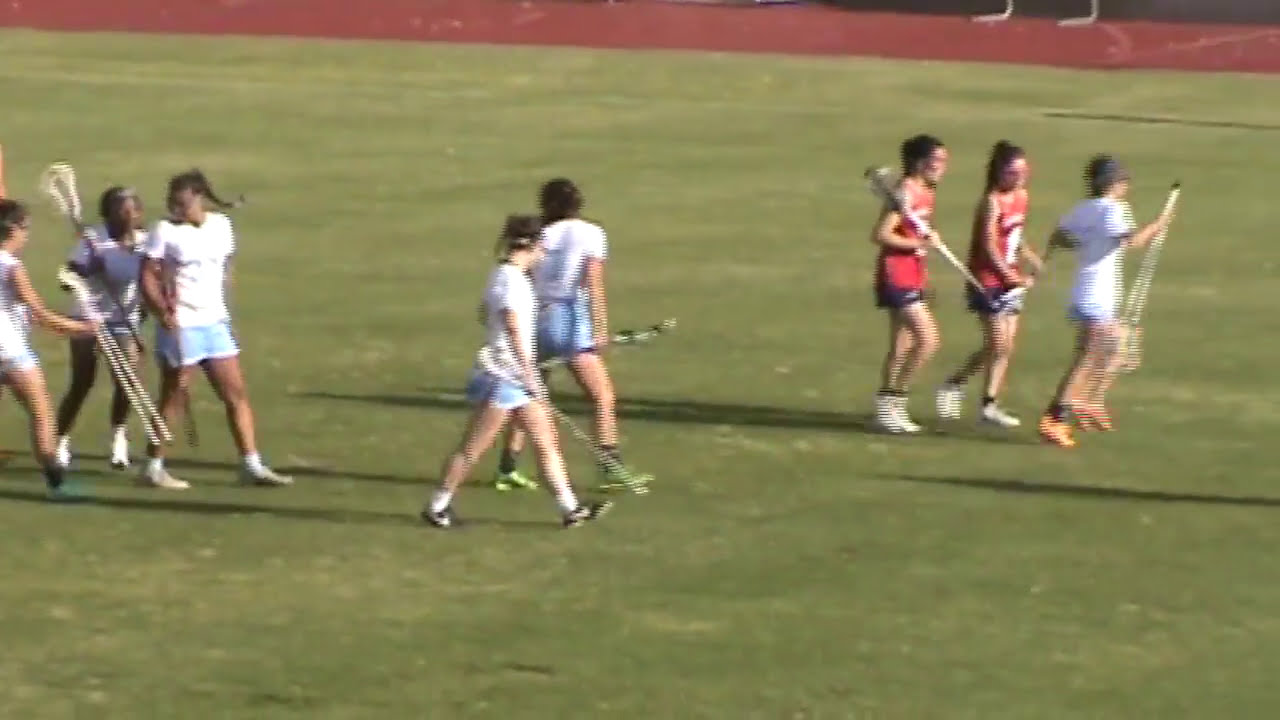An outdoor scene depicts a girls' lacrosse team on a grassy field, with short, green grass under the bright sunlight casting shadows to the left. The background shows a red border, likely a runner’s track. The image is overall blurry, obscuring finer details. The eight girls are arranged in three groups, moving from left to right. The three girls on the left, clustered together, are in white t-shirts and blue shorts, each holding a lacrosse stick. In the middle, two girls, similarly dressed in white and blue, walk in the same direction, with one looking back over her right shoulder. To the right, another cluster of three girls includes two in red shirts and blue shorts, and one in white. The girls are all wearing athletic shoes and have their hair tied up for the sport.